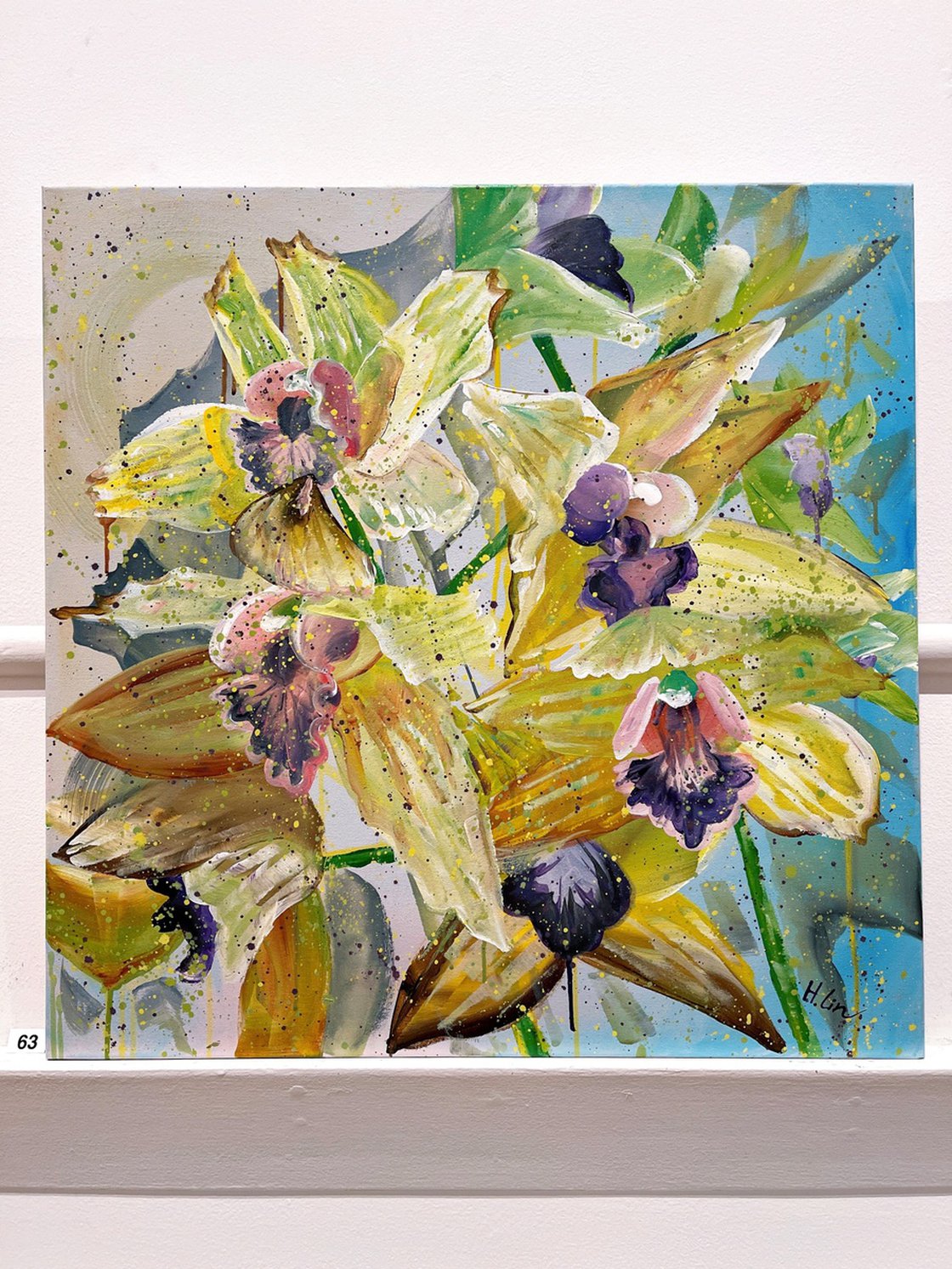This image captures a vibrant and richly detailed original square painting titled *The Dreamy Lovers* by artist Hisin Lin. The painting features a cluster of yellow cymbidium orchids with light purple centers and pink filaments, their creamy yellow petals creating a captivating visual centerpiece. The blooms, painted with either watercolor or oil paint, dominate the canvas and are connected by green stems. The background is divided with an aqua hue on the right and a pinkish beige on the left, accentuated by tiny speckles of dark paint splatters, enhancing the modern art aesthetic. The painting is set against a gray background and rests on a white ledge with a bar and wall, also white. In the bottom left corner, a small white tag bears the number 63. The overall composition features rich, vivid colors and dynamic details, encapsulating the beauty and allure of the floral subject.